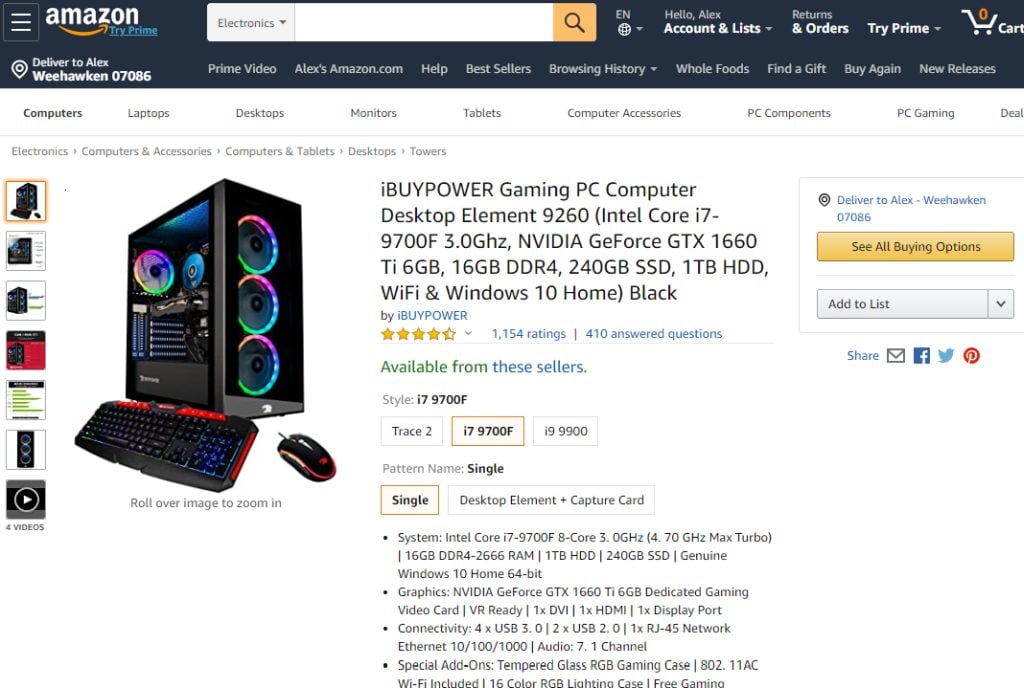The image depicts a product page from Amazon, showcasing an iBuyPower gaming PC desktop titled "Element 9260." The detailed product information reveals that the system is equipped with an Intel Core i7-9700F processor running at 3.0 GHz. Graphics capabilities are provided by an Nvidia GeForce GTX 1660 Ti with 6 GB of VRAM. Memory and storage specifications include 16 GB of DDR4 RAM, a 240 GB SSD, and a 1 TB HDD. Connectivity options include built-in Wi-Fi. The operating system is Windows 10 Home, and the entire setup is housed in a sleek, black chassis. The selected configuration under the 'Style' option confirms the Intel Core i7-9700F.